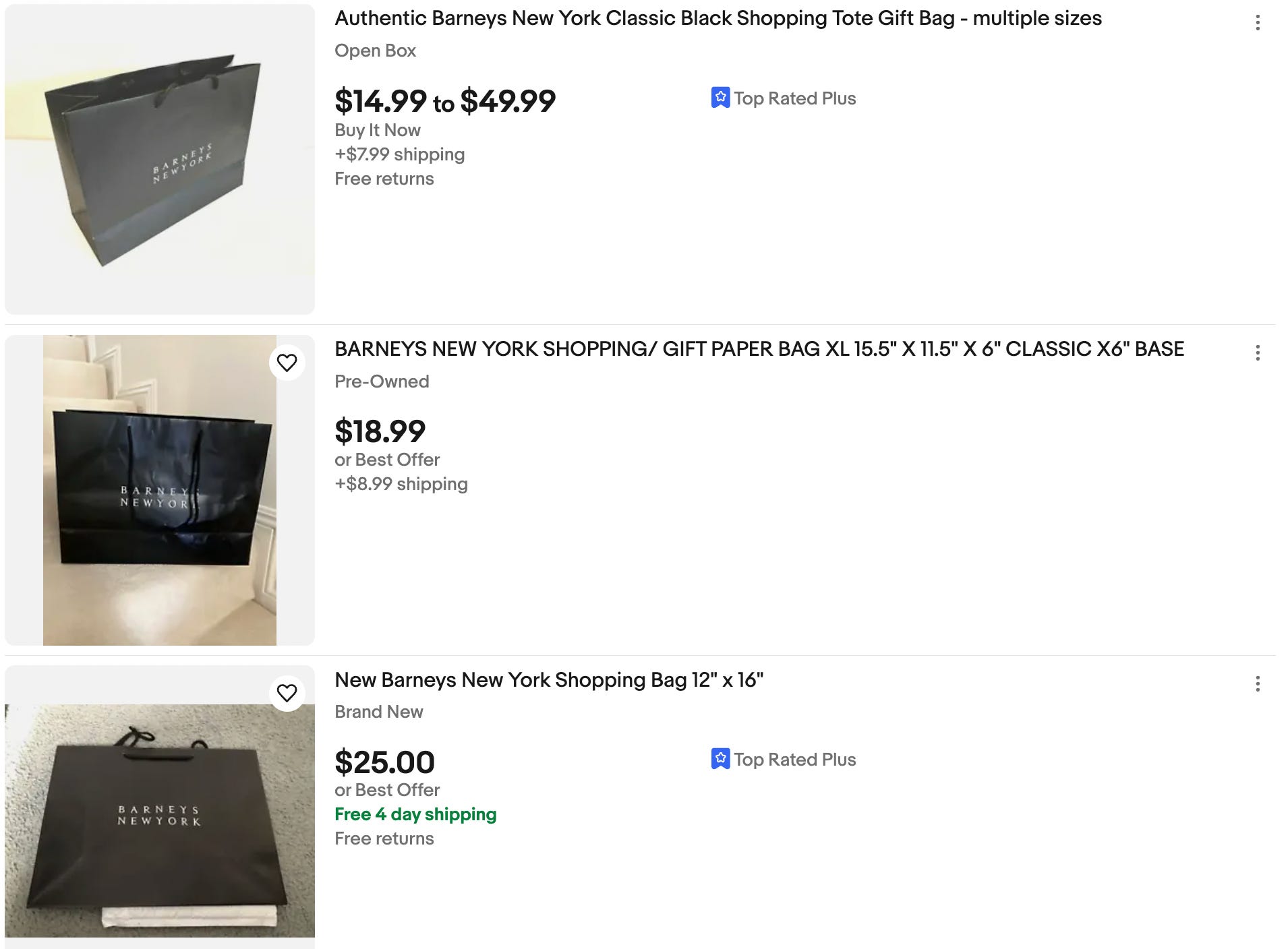This image captures three eBay-style product listings for black Barney's New York shopping totes. The listings are displayed vertically, each featuring a photo and detailed product information. The first listing depicts a black tote bag standing upright on a white background. It is described as an authentic Barney's New York Classic Black Shopping Tote gift bag, available in multiple sizes, priced between $14.99 and $49.99, marked as "top-rated plus," with a "buy it now" option, and $7.99 for shipping with free returns. The second listing showcases the same tote bag, this time displayed on a staircase, titled "Barney's New York Shopping/Gift Paper Bag XL 16.5x11.5x6," noted as pre-owned with a price of $18.99 or best offer and $8.99 shipping. The third listing features the bag laid flat, described as a new Barney's New York shopping bag, size 12x16, priced at $25 or best offer with free four-day shipping and free returns, also labeled "top-rated plus." Each listing highlights the distinctive Barney's New York branding on the bags.